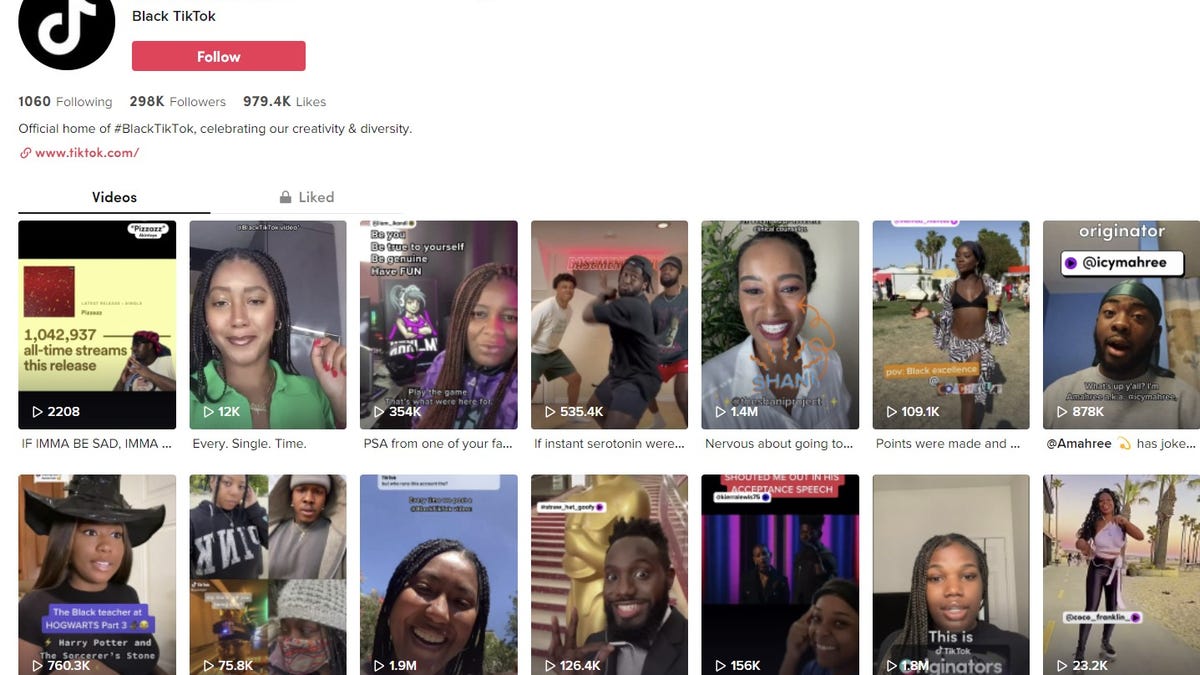**Descriptive Caption:**

This image showcases a screenshot from a website featuring a profile on TikTok. The background is predominantly white, with a partially visible logo at the top. Only the bottom half of the logo, which is a black circle containing a white letter "T," is shown. Adjacent to this logo is the text "Black TikTok" in two parts: "TikTok" appears in black with two capital "T"s, and "Black" follows as a separate word with a capital "B".

Beneath this, there is a prominent red banner featuring the white text "Follow." The profile statistics are displayed below: "1060 following," "298K followers," and "979.4K likes." It also indicates that this is the "Official home of #BlackTikTok," celebrating creativity and diversity.

The screenshot provides the TikTok web address and includes two main sections labeled "Videos" and "Liked." "Videos" is underlined in black, while "Liked" is marked with a padlock icon. Below this, there are two parallel rows, each containing seven panels. The panels feature a variety of images or video thumbnails, most of which include people and their usernames.